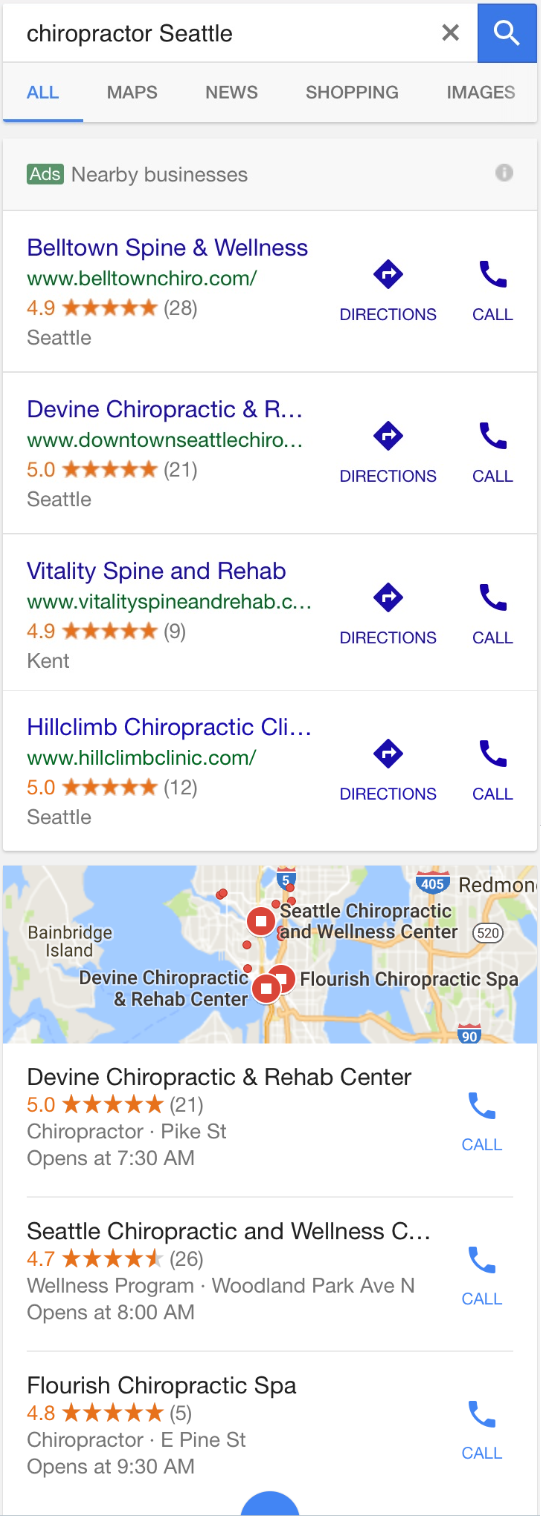This image appears to be a screenshot from a mobile device, likely a smartphone or tablet, evident from its aspect ratio. At the top, there is a search box featuring a blue magnifying glass icon. Immediately below the search box, there are various tabs for different search categories—All, Maps, News, Shopping, and Images—with the "All" tab currently selected. Following the tabs, the image displays targeted advertisements and listings for nearby businesses. 

The focus of the image is on search results for "Chiropractic Seattle," showcasing various chiropractic practices in the area. The first listing is for "Belltown Spine and Wellness," which has a 4.9-star rating based on 28 reviews and is located in Seattle. Next is "Divine Chiropractic," with a perfect 5-star rating from 21 reviews, also in Seattle. Following that is "Vitality Spine and Rehab" in Kent, boasting a 4.9-star rating from 9 reviews. "Hill Climb Chiropractic" in Seattle also holds a 5-star rating from 12 reviews. Another listing for "Divine Chiropractic and Rehab Center" in Seattle shows the same 5-star rating and 21 reviews. "Chiropractic and Wellness" has a 4.7-star rating from 26 reviews, and "Flourish Chiropractic Spa" has a 4.8-star rating from 5 reviews.

The listings are accompanied by a map pinpointing these locations with icons, highlighting the Seattle metropolitan area. Each business entry includes options for "Directions" and "Call" to facilitate easy navigation and contact. This detailed listing underscores a Google search query for chiropractic services in the Seattle area.